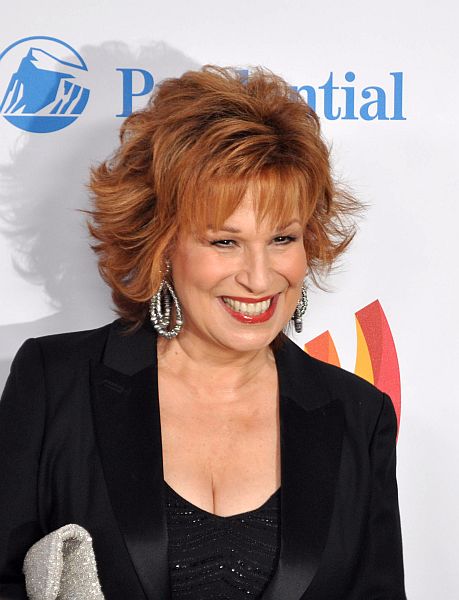In the picture, there is a well-dressed woman who appears to be a celebrity, standing in front of a large white banner with "Prudential" written in blue and a blue emblem resembling a mountain or iceberg. The woman, who looks to be in her 40s or 50s, has long, reddish-orange hair with bangs and is wearing noticeable makeup, including red lipstick. Her outfit consists of a black suit jacket over a low-cut black top adorned with sequins or sparkles, revealing a hint of cleavage. She accessorizes with large, sparkly, oval-shaped silver earrings, and she is holding a small, shiny silver clutch under her arm. The background includes various advertisements, partially covered by her figure, and a shadow cast by the camera flash on the banner. The woman has a wide, toothy smile and is looking slightly away from the camera. She appears to have a normal body weight, balanced and confident in her presence.